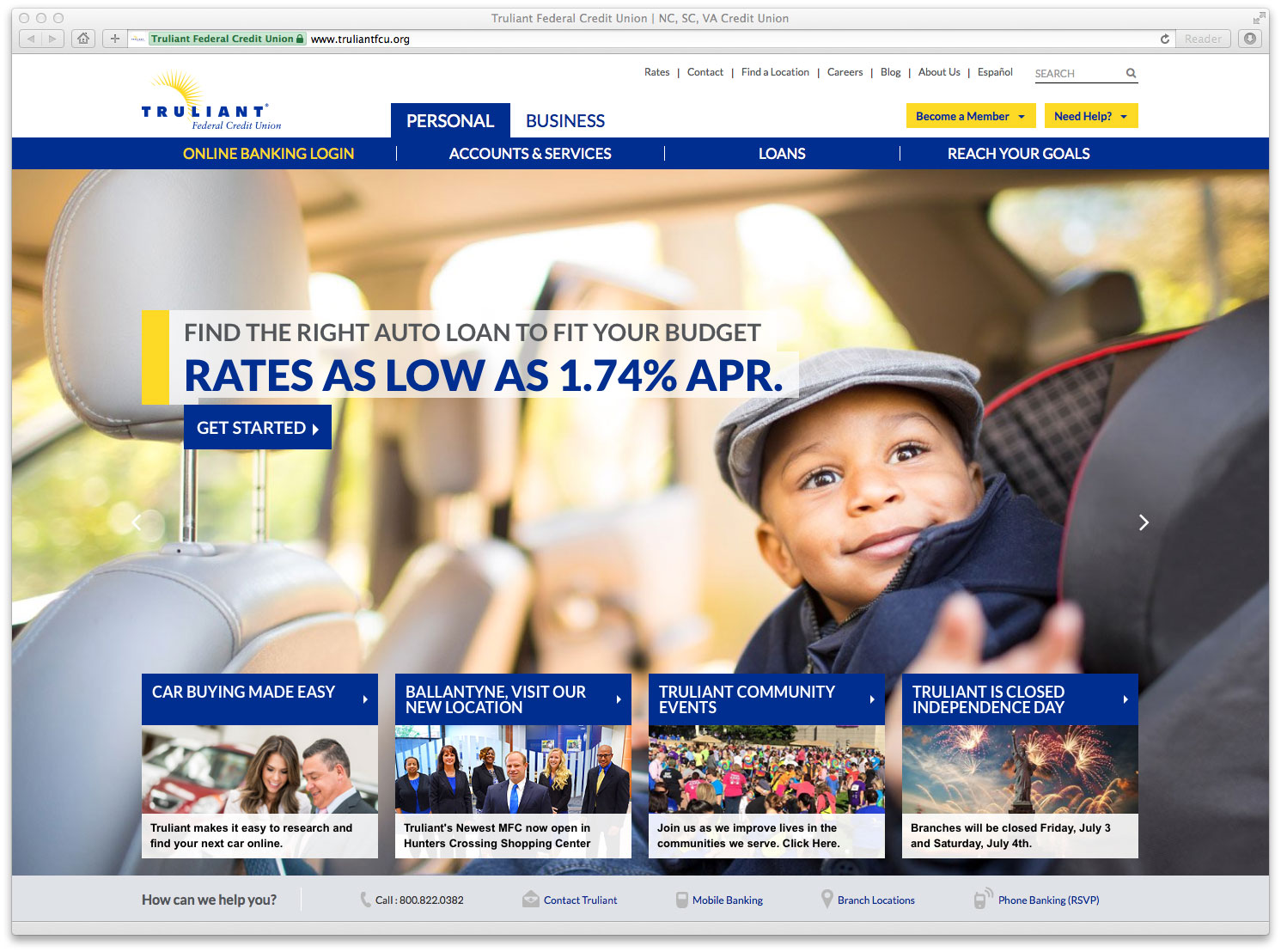The website interface displays a top section with a light gray background featuring three circles suggesting the use of an Apple device. In the center of this section, in dark gray text, it reads "TrueLion Federal Credit Union" followed by "NC, SC, VA Credit Union". 

Below this, the web browser interface is white with a gray outline. On the left, in a green rectangle with green font, it states "TrueLion Federal Credit Union" alongside a lock icon. Adjacent to this, the website URL is displayed in black: www.truelionfcu.org.

The main content area of the webpage has a white background. In the upper left-hand corner, "TrueLion Federal Credit Union" is written in blue. The navigation menu on the right includes tabs labeled in black: Raise Contact, Find Location, Careers, Blog, About Us, Español, and Densest Search Online.

Below these tabs, there are two yellow buttons with blue text: "Become a Member" and "Need Help". Additional tabs, including “Online Login” (in yellow text), “Accounts and Services”, “Loans”, and “Reaching Goals” are found beneath.

Further down, there is an image of a child in a car seat. The child, dressed in a blue jacket and an old-style gray newspaper hat, is smiling and has brown eyes. The photo captures the moment of the child’s delight, presumably directed at a parent who is engaging with him.